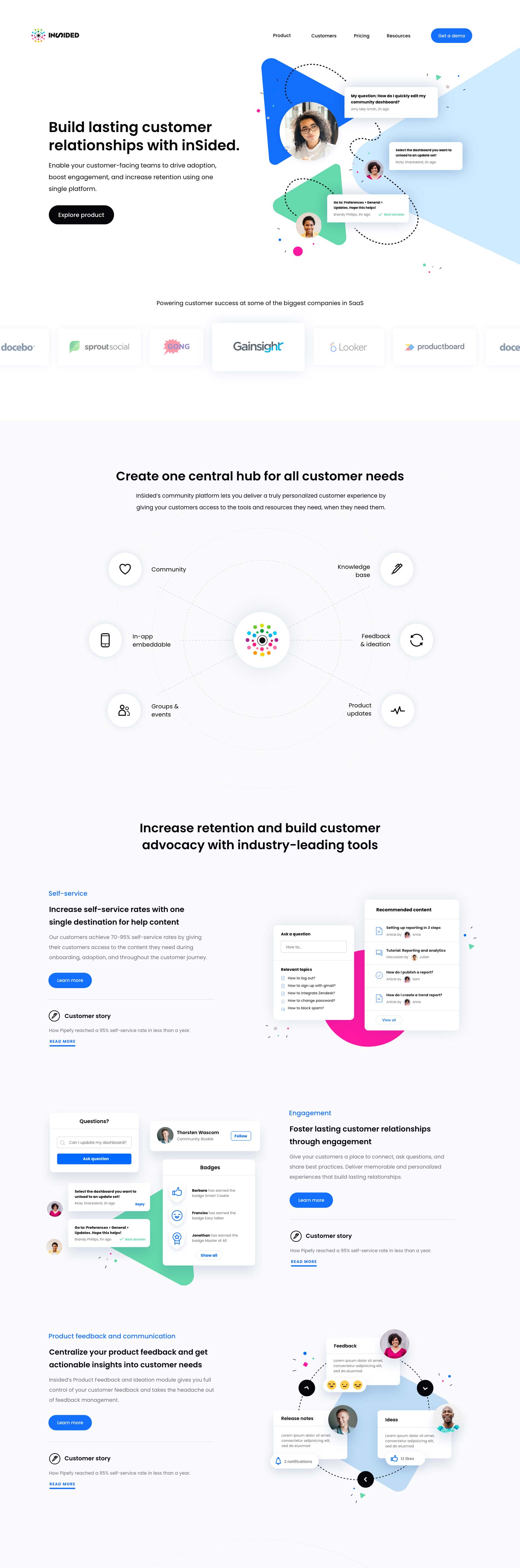The image is a detailed promotional capture from the website "Insighted." The webpage prominently features the company's logo, where "Insighted" is written with a distinct design: the 'S' is capitalized and turned sideways, while the rest of the letters are in lowercase. In the icon at the top, the entire name is in uppercase with the 'S' uniquely rotated.

The primary message conveyed is, "Build lasting customer relationships with Insighted." Below this headline, additional text emphasizes the platform's capabilities: "Explore product, enable your customer-facing teams to drive adoption, boost engagement, and increase retention using one single platform." 

The image also includes visuals of interconnected people, joined by a dotted line, with abstract triangles in the background for a modern and dynamic design. Further down the page, there's a section titled "Create one central hub for all customer needs," featuring categories like Community, In-App, Embeddable, Groups and Events, Knowledge Base, Feedback and Ideation, and Product Updates.

A subsequent section reads, "Increase retention and build customer advocacy with industry-leading tools." Here, a couple of rectangles contain more detailed information, each accompanied by a highlighted "Learn More" button. Additional segments of the webpage include further detailed content, enhancing the user’s understanding of Insighted’s offerings.